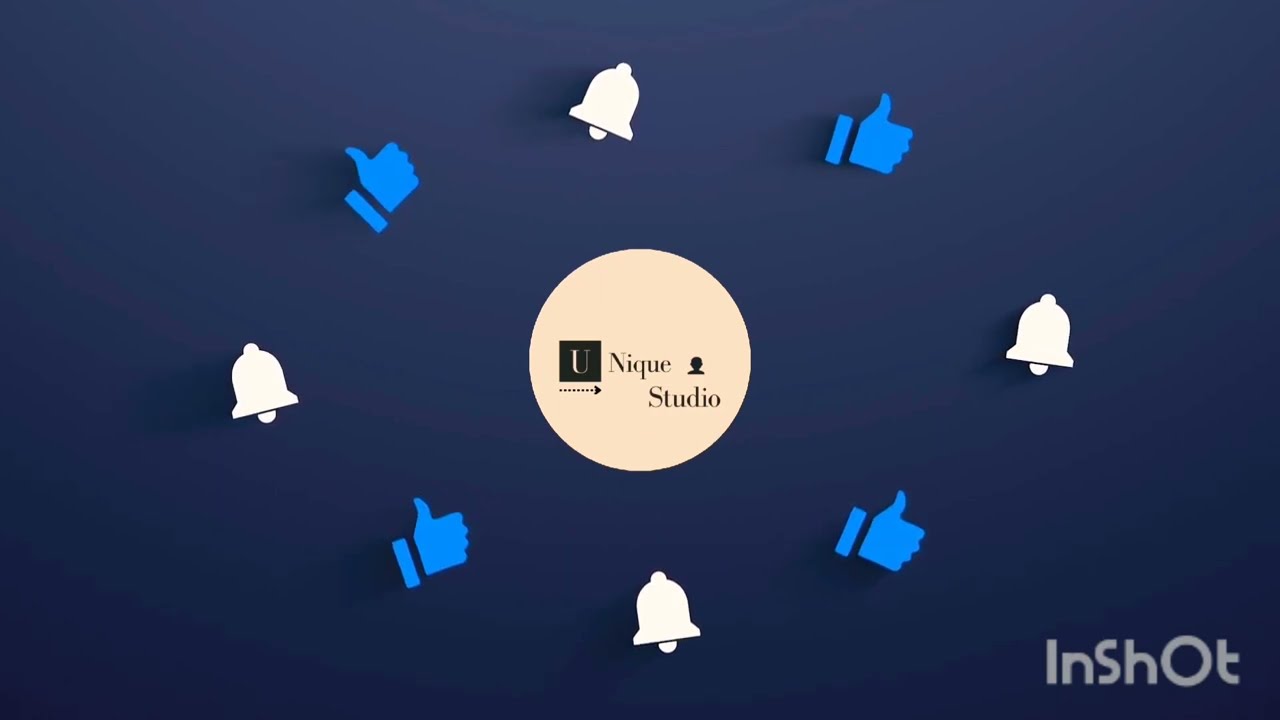This high-definition, wide photograph features a central white circle positioned against a textured navy blue background. Encircling the central design, the white circle contains the text "Unique Studio" in black letters, with a distinct 'U' displayed in white lettering inside a black square. Additionally, a silhouette of a head in black is positioned above the word "Studio" within the circle. Surrounding this central circle are alternating cut-out images of blue thumbs-up hands and white bells, creating a patterned border. The lower right corner of the image contains the name "InShot" in white letters, with a stylized mix of uppercase and lowercase characters.